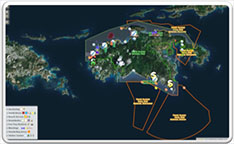The image depicts an extremely small and detailed map, possibly of an island located near regions like New Zealand or Southeast Asia. The primary focus is on a prominent island dotted with numerous tiny icons and labeled with text in yellow or light green, which are too small to read clearly. Surrounding this main island are several smaller islands, particularly visible to the left and top of the primary island, with the lower part of the image dominated by dark blue sea. Red lines demarcate certain sea areas adjacent to the island, indicating specific boundaries or zones. The map also includes a legend in the lower left corner, further adding to its detailed portrayal of the island's physical features and labeled elements.